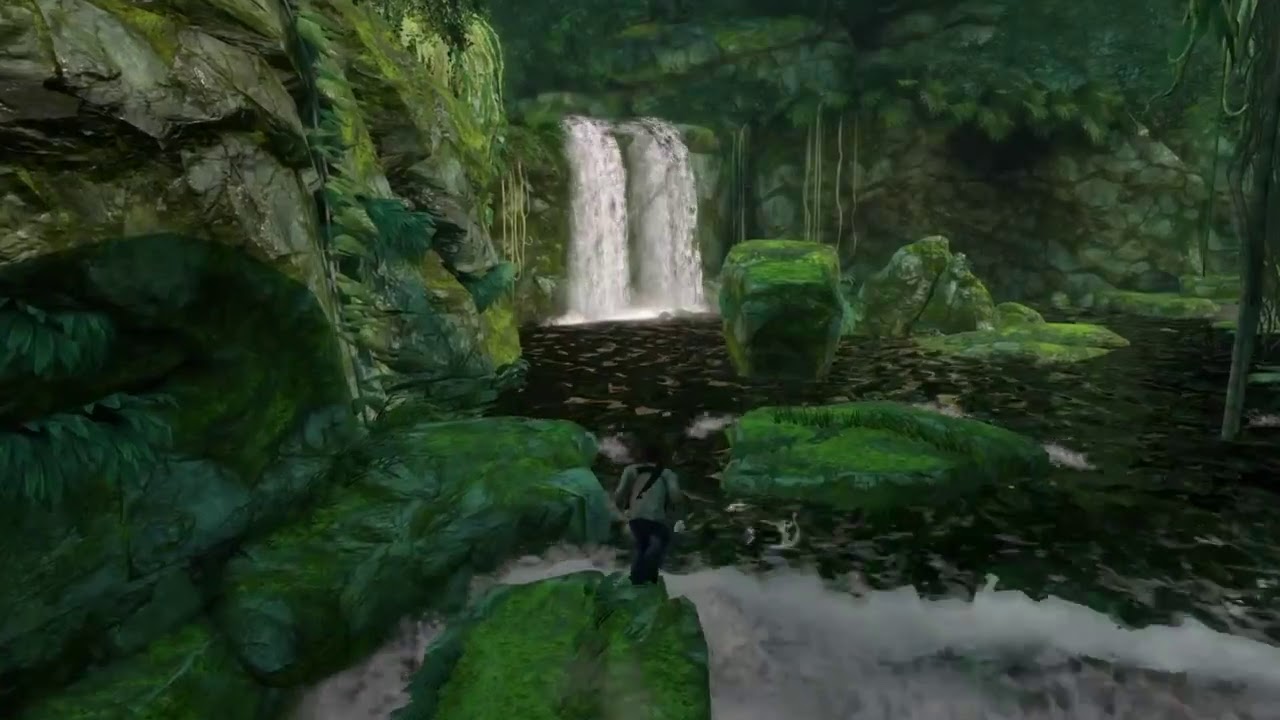The image depicts a striking and picturesque waterfall, possibly enhanced with a filter or displaying exceptional natural beauty that makes it appear somewhat unreal. The centerpiece is a twin-segment waterfall, approximately 30 to 40 feet tall, pouring into a dark, possibly crystal-clear pool with black and brown rocks underneath. Surrounding the scene are towering vegetated rock walls adorned with thick, lush greenery, extensive vines, and patches of exposed brown rock. A person stands prominently in the foreground on a green-tinted rock, facing the waterfall. The individual is dressed in a green shirt and blue jeans, with what appears to be a semi-automatic rifle on their back, suggesting they are a character from a high-definition video game. The scene is encapsulated by the verdant wilderness, creating a sense of solitude and adventure, as the pool's white water churns and rushes further downstream.